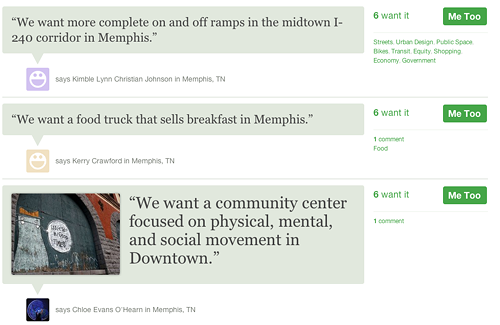In a lively public forum focused on urban development in Memphis, Tennessee, local residents expressed their diverse needs and hopes for the community. Kimby Lee Christian called for more comprehensive on-and-off ramps in the Midtown I-240 corridor to improve accessibility. Mary Croswell voiced her desire for a food truck offering breakfast options to cater to the morning rush. Chode Evans O'Harm advocated for a community center in downtown that emphasizes physical, mental, and social well-being.

The discussion highlights the intersection of urban design, public space, and community needs, covering topics like bikes, transit, equity, shopping, and local economy. Despite the varied concerns, one voice diverged to express a deeply personal perspective on spirituality and religious faith, underscoring the diversity of opinions within the community. The forum painted a vivid picture of a city grappling with change, aiming to balance modernization with preserving the community's core values.